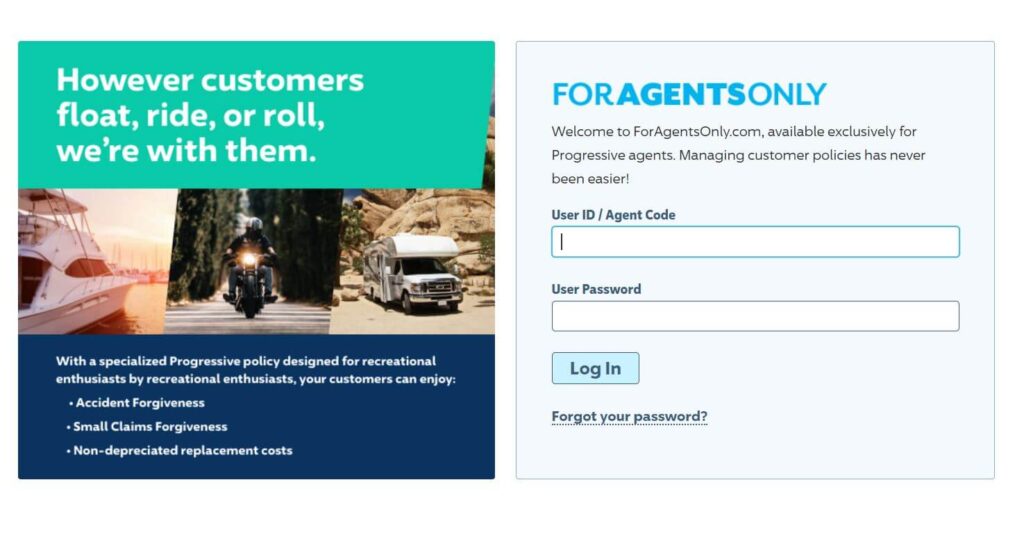This image is a cropped screenshot from a web page, showcasing two distinct square sections placed side by side. The first section features an image with graphical text overlays, encapsulated primarily in rectangular boxes. At the top of this section, a green rectangle contains a message in white text: "However customers float, ride, or roll, we're with them." Below this, three images are arranged side by side, depicting different recreational vehicles—a yacht, a motorbike, and a motor caravan. Further down, a dark blue rectangle offers additional information about small claims and accidents for recreational users, providing supportive text in a contrasting font.

The second section to the right is a light blue square dedicated to user authentication. This part includes fields for User ID and User Password, accompanied by a prominent blue login button below. Additionally, a hyperlink is provided for users who may have forgotten their password, facilitating easy recovery.

The overall design focuses on providing information and user interaction, structured neatly within a cropped screenshot format that excludes navigation, menu buttons, and other web browser elements.